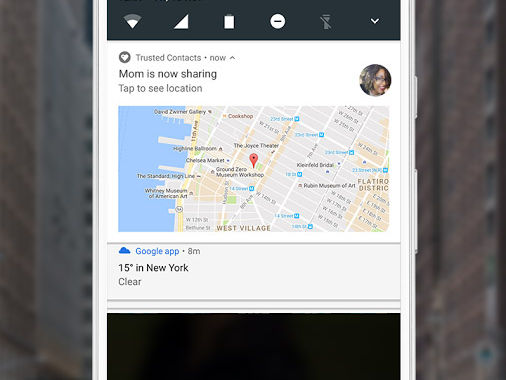The image is a screenshot of a smartphone displaying a location-sharing notification. At the top of the screen, a black bar includes icons for Wi-Fi signal, phone signal strength, battery level, a "Do Not Disturb" symbol, and a flashlight that is turned off. A drop-down menu is also visible within this bar.

The main screen has a notification from the "Trusted Contacts" app in white text, indicating that "Mom is now sharing." A prompt suggests tapping to view the location. To the right of this notification is a small avatar image of the mother, depicting an African woman with curly or braided hair.

Below the notification, there is a map with a red pin, suggesting the location is in the West Village area, near the Joyce Theater or Ground Zero Museum Workshop. Additionally, a Google app notification from eight minutes ago reports that the temperature in New York is 15 degrees. There is an option to clear this weather notification.

The entire screenshot is displayed within the rendering of a phone. The background image is blurred, showing city buildings but lacking discernible details. The primary focus of the image is on the "Trusted Contacts" notification signaling the shared location.